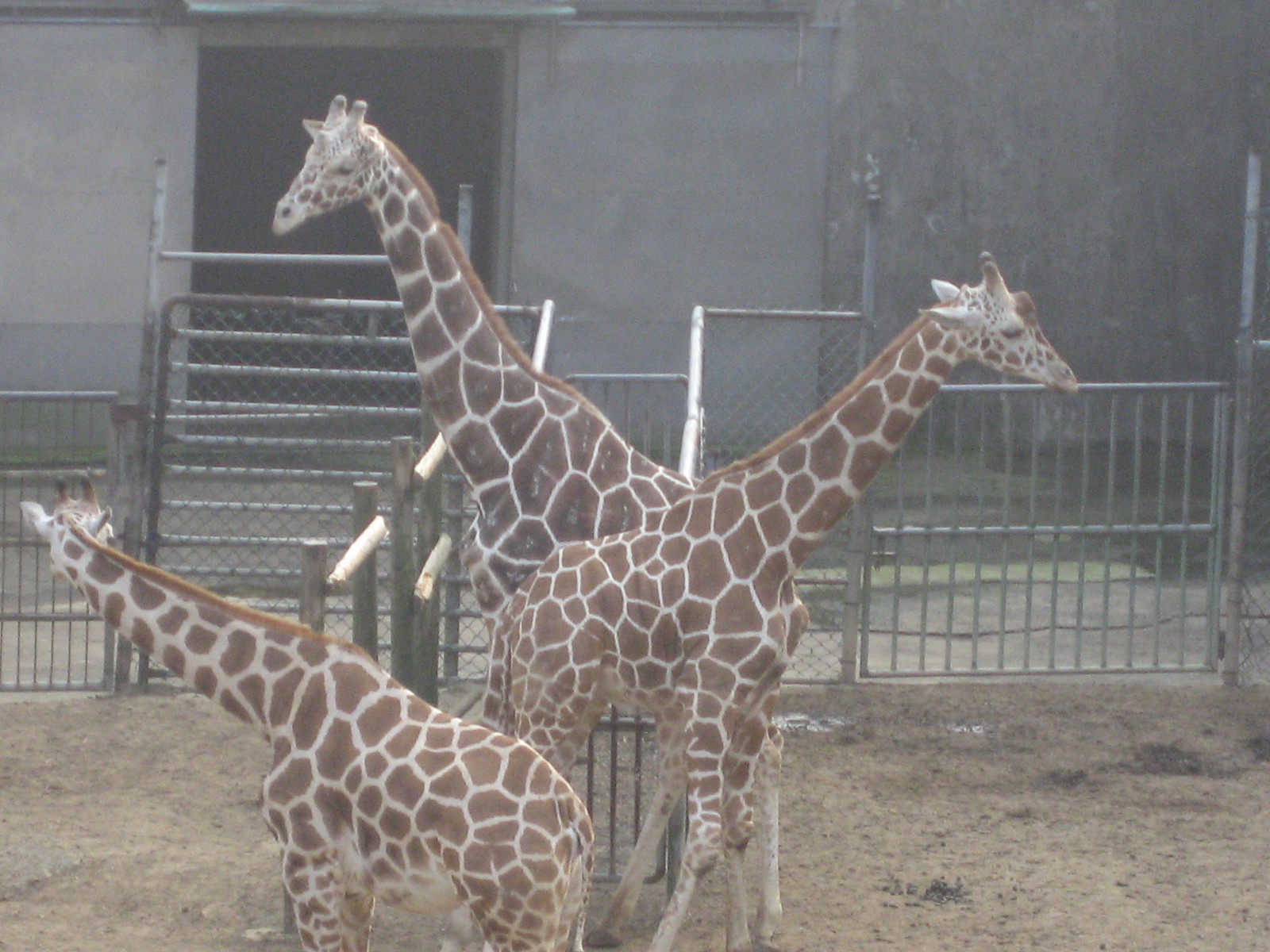This outdoor photograph features a trio of giraffes in a fenced enclosure comprised of wire and chain-link materials. The setting appears to be either early morning or a cloudy day, as suggested by the soft, almost grey light that bathes the scene. In the foreground, the giraffes stand on a terrain of light-colored dirt and soil. The three giraffes vary in size, with two adults and a younger one, arranged horizontally. The giraffe closest to the viewer faces left, the one in the middle faces right, and the giraffe farthest back also faces left.

In the background, a grey outbuilding with a large, open door casts deep shadows that obscure the interior, while a paved cement walkway lies directly in front of this structure. The animals are confined within an enclosure delineated by metal gates and railings. Each giraffe looks in a different direction, creating a dynamic composition. The simplicity of the scene focuses attention on these majestic creatures and their varied stances.